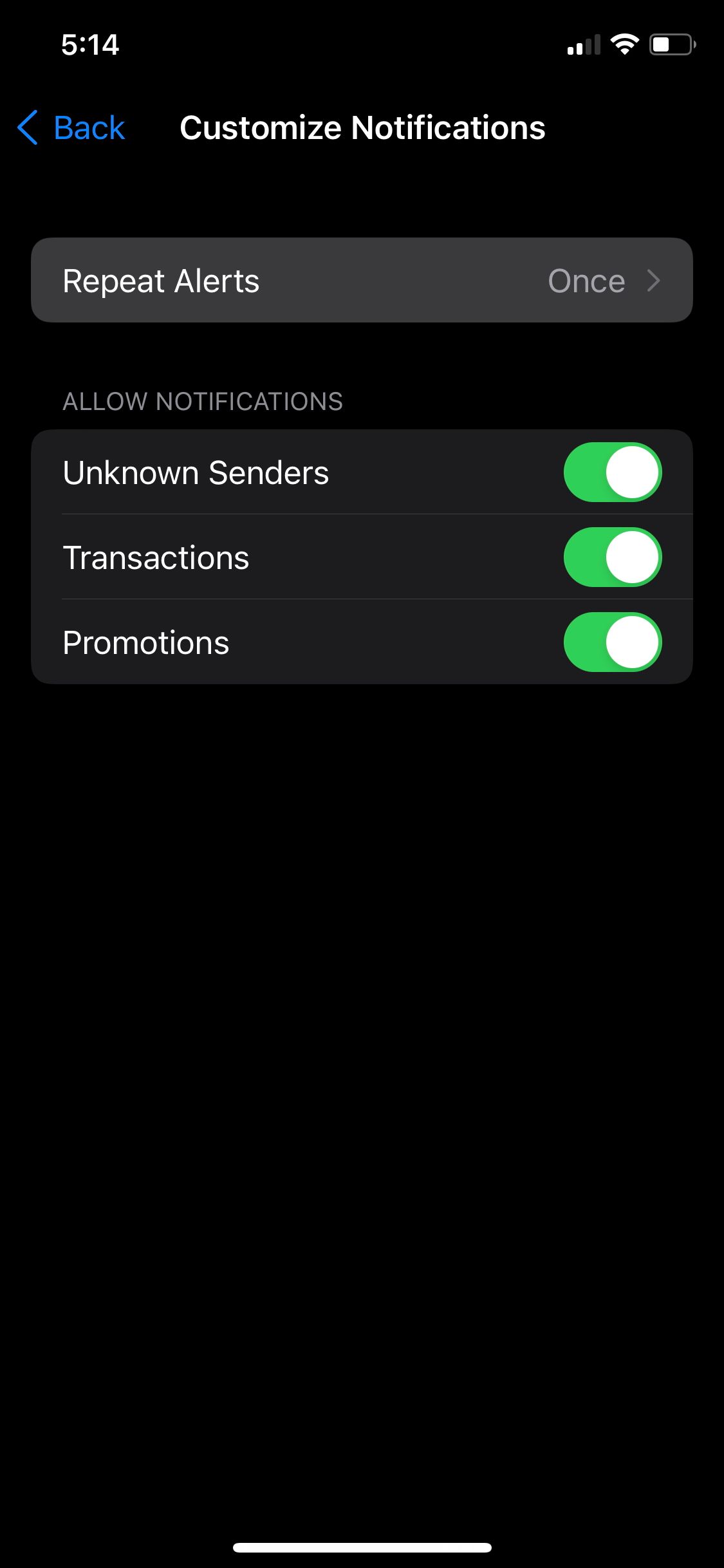The image depicts a long black rectangle, resembling a smartphone screen, filled with various settings and notifications. In the upper left-hand corner, the number "514" is displayed in white lettering. Below this, "BAC" is written in blue letters, accompanied by a blue arrow pointing to the left. To the right, the text "Customized Notifications" appears in bold white lettering. 

At the top of the screen are the typical status indicators: phone signal bars, Wi-Fi signal, and a battery icon showing it's halfway charged. Beneath "Customized Notifications," a gray rectangle stretches horizontally with the text "Repeat Alerts" in white on the left, and "Once" on the right, accompanied by a light gray arrow pointing to the right.

Further down, the text "Allow Notifications" is written in gray. Below this section, "Unknown Senders" is displayed in white lettering on a grayish background. To its right is a green circle featuring a smaller white circle inside, positioned to the right, indicating a toggle switch.

Below "Unknown Senders," the word "Transactions" appears in white lettering, with a similar green circle and white toggle switch to the right. Lastly, "Promotions" is also shown in white, paired with the same green and white toggle switch. At the very bottom of the screen, a white bar spans from left to right.